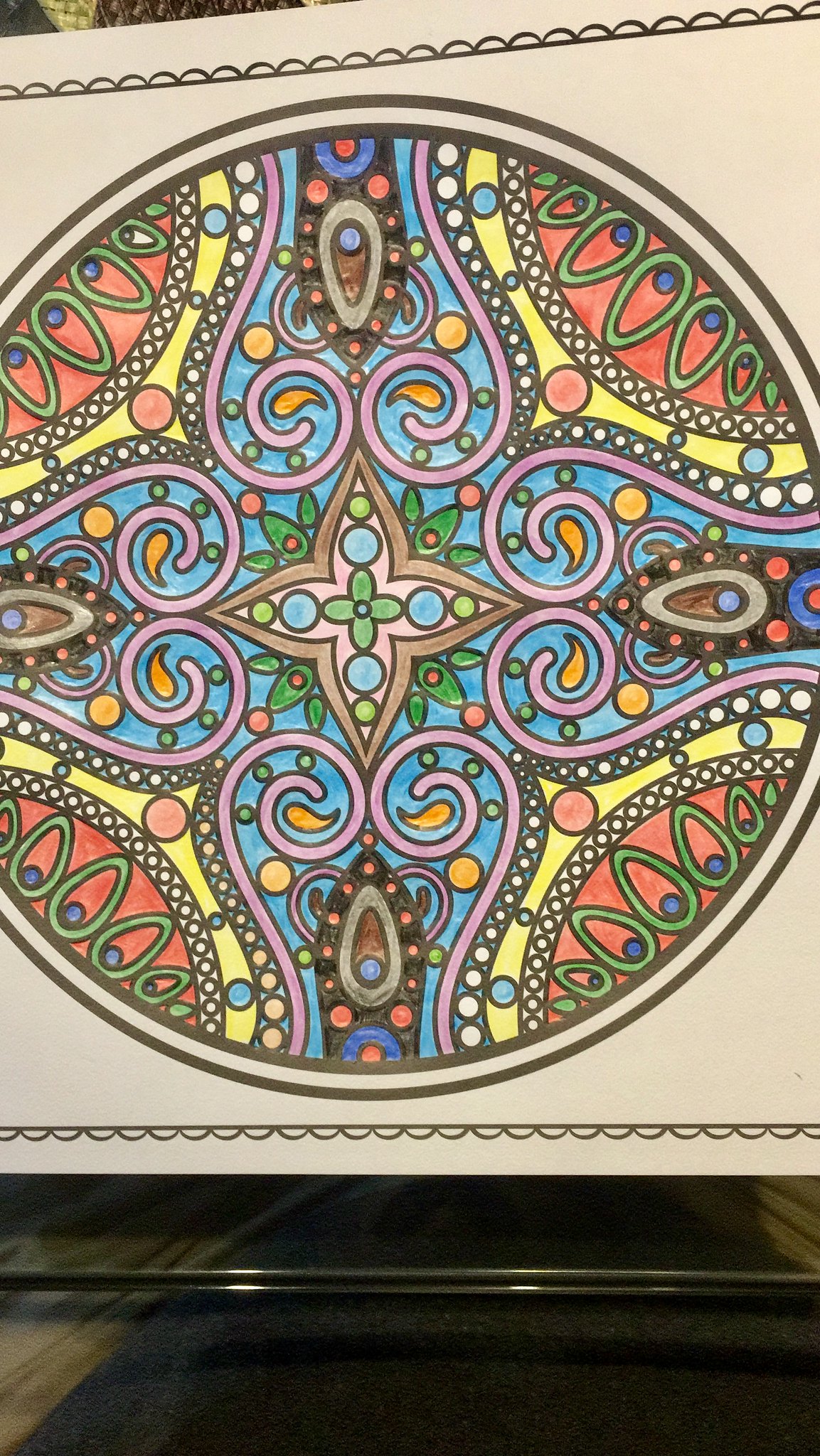This image features a meticulously colored mandala, resembling a page from an adult coloring book. The artwork is crafted on pristine white paper, bordered by a clear white frame, and is set against a black fabric table or cabinet. The circular mandala is adorned with intricate geometric swirls. At its core, a four-part flower design is elegantly detailed with green leaves extending from each of its corners. Each flower petal culminates in a curved, heart-like shape, predominantly colored in a deep purple hue, intricately decorated with green and orange dots.

Central to these heart-shaped sections is an elegant peacock tail-like protrusion, contributing to the mandala's detailed and elaborate aesthetic. The color palette predominantly features rich reds, a dominant blue background, and vibrant yellow accents that delineate various components of the design. Interspersing the geometry are striking black lines with black circles that further define the structure of the mandala. Encircling the outer edge are green, egg-shaped figures, each dotted with blue, creating a harmonious frame around the entire mandala.